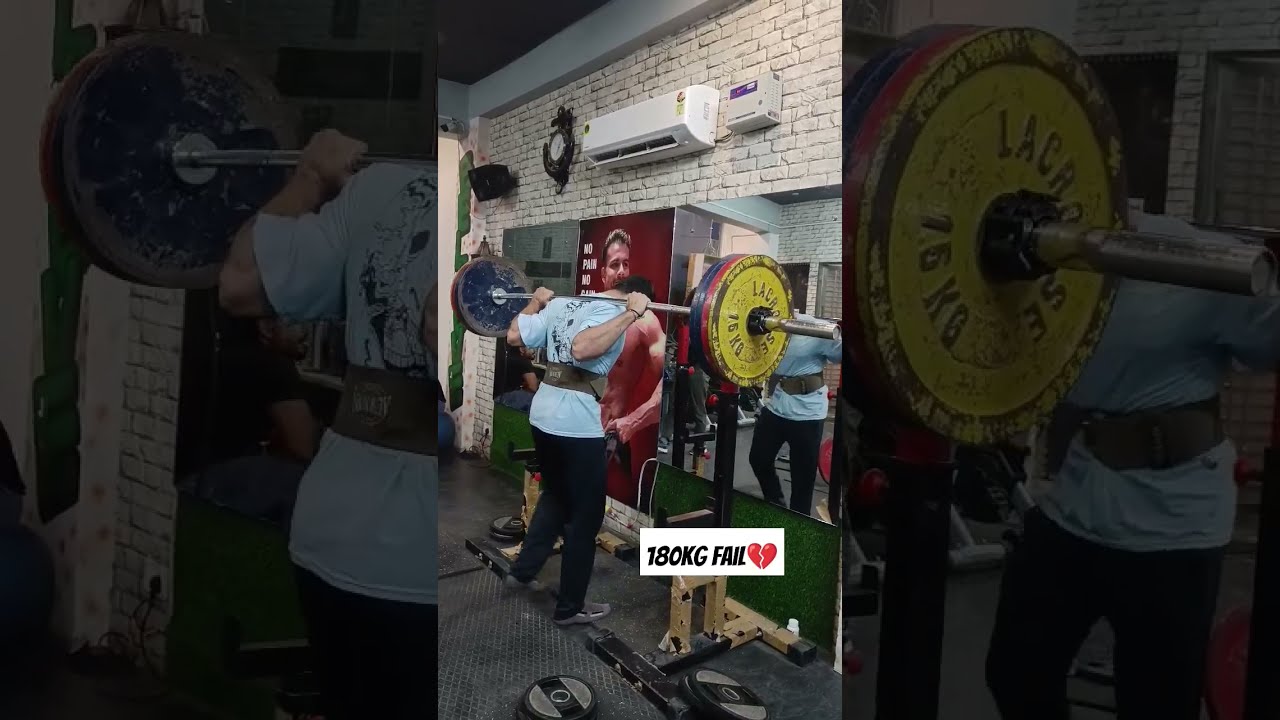In this image, we see a detailed scene set in a weight training room or gym, captured in a horizontal rectangular frame divided into three equal panels. The central focus of the image is a man standing directly in the middle, holding a large barbell with weights positioned on his back at shoulder level. He is clad in a light blue t-shirt displaying some writing on the back, black slacks, and grayish sneakers, and he is secured by a weightlifting belt. The man is captured in front of a mirrored wall, reflecting his image, though the barbell obstructs his face in the reflection. 

The gym's floor is covered with a gray rubber mat, and the setting suggests that the man is lifting the weights from a pedestal. Above the mirror, the wall is constructed from exposed brick. There is green astroturf in front of the mirror with some posters visible to the left, including a red poster featuring a muscular man, though partially obscured by the lifter.

The image includes an overlay text at the bottom left stating "180 kg fail" in black against a white rectangle, accompanied by a cracked heart icon. This text implies the man might be attempting to lift 180 kg unsuccessfully. The left and right panels of the image are darker and focus on different segments of the scene. The left panel shows part of the man's left side, while the right panel contains a close-up view of his left-hand side reflected in the mirror. The entire composition, with its diverse color palette featuring tan, off-white, white, black, yellow, red, gray, and light blue tones, has a style reminiscent of a screenshot from TikTok or Instagram.